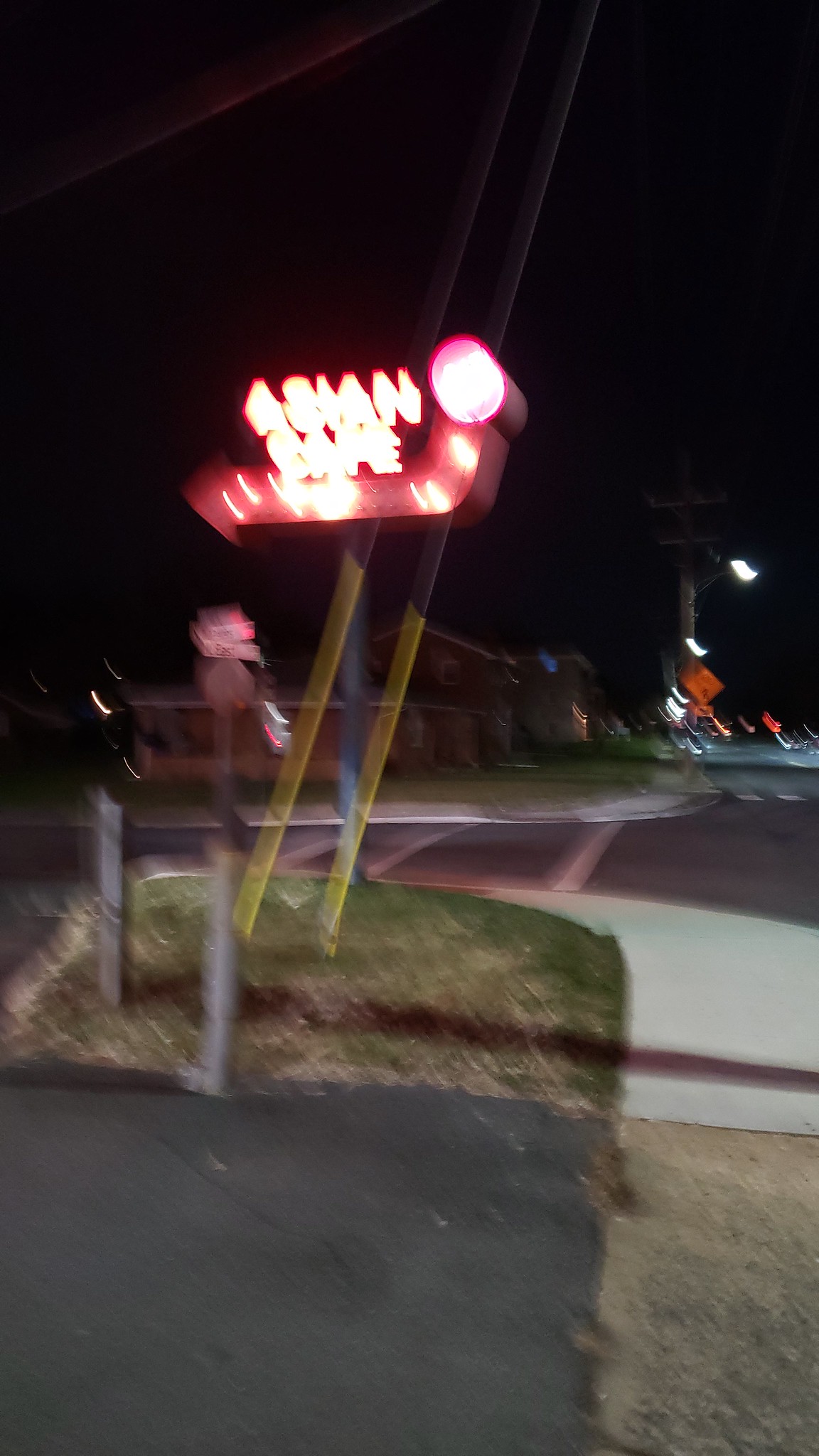In this nighttime image, we observe a street corner scene with a distinct urban atmosphere. The image is rather blurry, making some details challenging to discern. Dominating the scene is a large rectangular sign that reads "Asian Cafe" in bright, neon white letters with a red outline. Below the text, there's a prominent red arrow pointing to the left. This sign is positioned at the corner of the road, standing out against the dark sky.

The street itself features a dark gray concrete patch on the left and a light brown dirt patch on the right, transitioning into a grassy area. Two rods, which start off yellow and then turn gray, are visible and lead towards a lighter gray sidewalk, followed by a gray road marked with three horizontal white lines. Across the road, there is a red brick building set against a backdrop of green grass. Near this building, an orange diamond construction sign is mounted above a phone pole.

On the closer corner to the viewer, we can see part of a parking space and sidewalk, accompanied by several poles protruding from the ground. Despite the blurriness, the overall scene is illuminated by streetlights, highlighting the surrounding grass patches and other signs along the road.